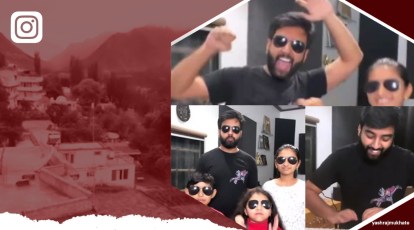The image consists of a rectangular horizontal frame with a rough, torn-off bottom left edge. The left 40% features a sepia-toned aerial photograph of a town, highlighted by buildings and a hillside. A red filter partially overlays this section. The right 60% holds a hexagonal white-bordered frame displaying three color photographs of the same man. The top photo shows the man, who has black hair, a beard, and dark sunglasses, wearing a black t-shirt with his hands raised and mouth open. A woman with dark sunglasses is partially visible beside him. The bottom left holds a family portrait: the same man, the same woman, and two children, all in sunglasses. The bottom right captures the man alone, without sunglasses but still in the black t-shirt. In the upper right corner, a white Instagram logo is present.